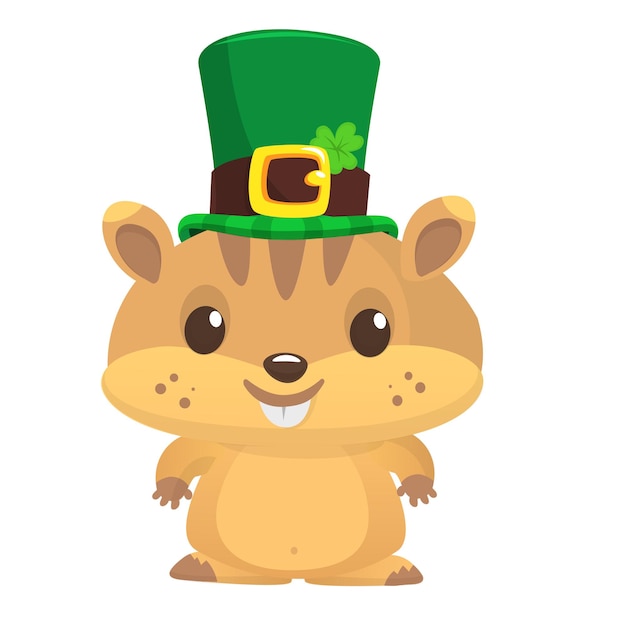This image features a cartoon figure of an animated animal, likely a chipmunk or perhaps a hamster, set against an all-white background. The character has a distinctive large head with a top half in light brown and a bottom half in light tan. It has a single white tooth protruding from its smiling mouth, giving it a somewhat nerdy appearance. The character has black eyes, light brown freckles on the lower face, and ears that are outlined in light brown and tan with a darker brown middle. This chipmunk is adorned with a festive green leprechaun hat that features a brown leather belt with a gold buckle and a green four-leaf clover, fitting a St. Patrick's Day theme. The body of the chipmunk is small relative to its head, with short arms and legs, and the legs face sideways. Overall, the chipmunk appears cheerful and ready to celebrate.